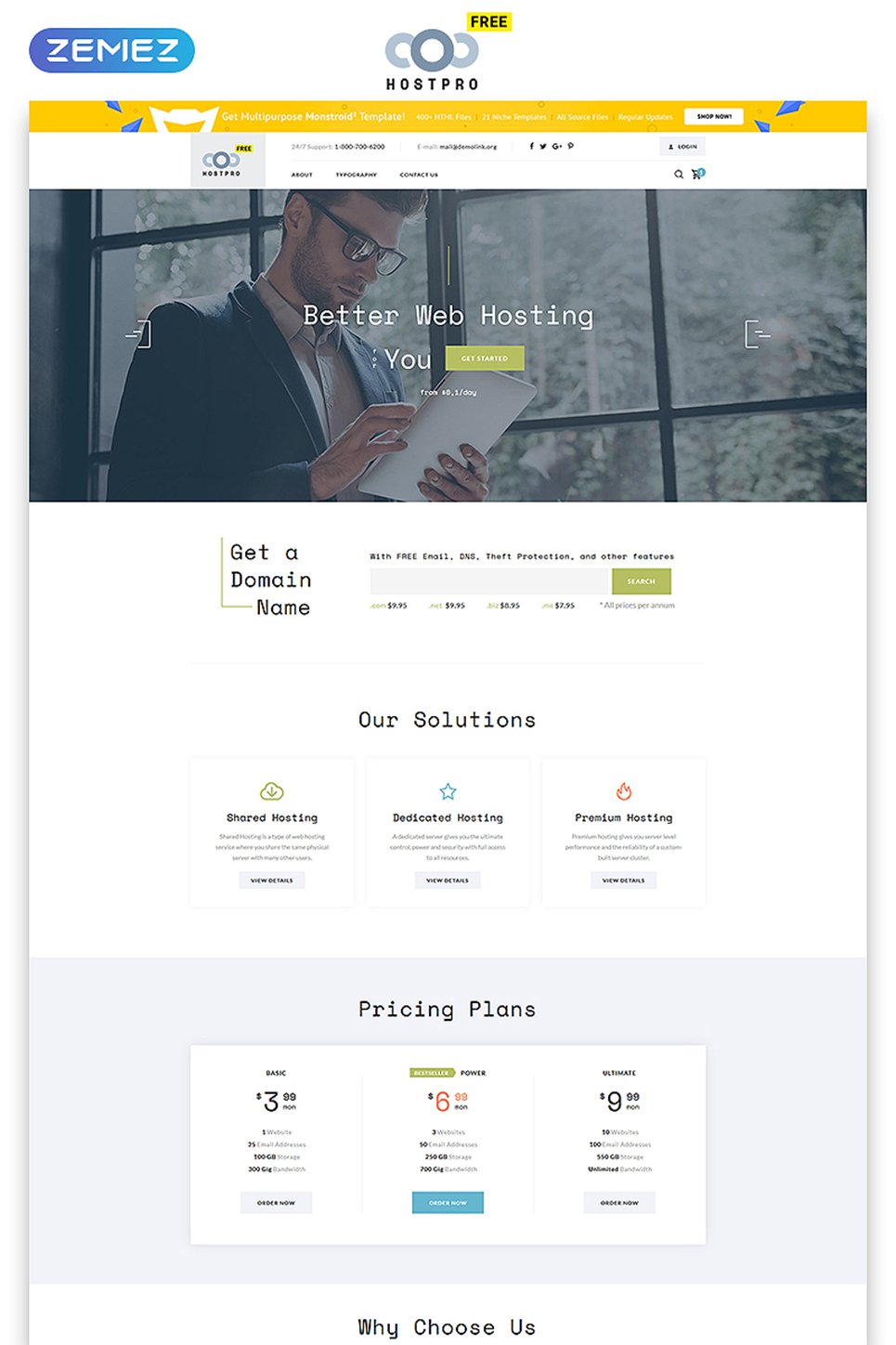The image showcases a section of the Zemez website, a company specializing in hosting solutions. The logo features an oval-shaped design with a blend of blue and turquoise colors. Prominently displayed in the center of the webpage is the title "Host Pro," surrounded by four gray circles, one of which highlights the word "Free."

A striking gold bar runs horizontally across the section, accompanied by a white bar beneath it. Towards the top of the page, there is a search bar for users to find specific content. Adjacent to this search bar, an image depicts a man gazing down at a clipboard or laptop. He is characterized by his glasses, beard, mustache, and brown hair. He wears a suit jacket over a gray button-down shirt.

The webpage invites users to "Get a Domain Name" with a prominently displayed search bar for entering domain information. Below this section, the site introduces their various hosting solutions: "Shared Hosting," "Dedicated Hosting," and "Precision Hosting." Though each option includes additional details, they are small and not easily readable.

In a more prominent gray box, a white inset provides information about pricing plans, highlighting three tiers: $3.99, $6.99, and $9.99. Towards the bottom of the page, there is a clickable section titled "Why Choose Us," offering further details to potential customers.